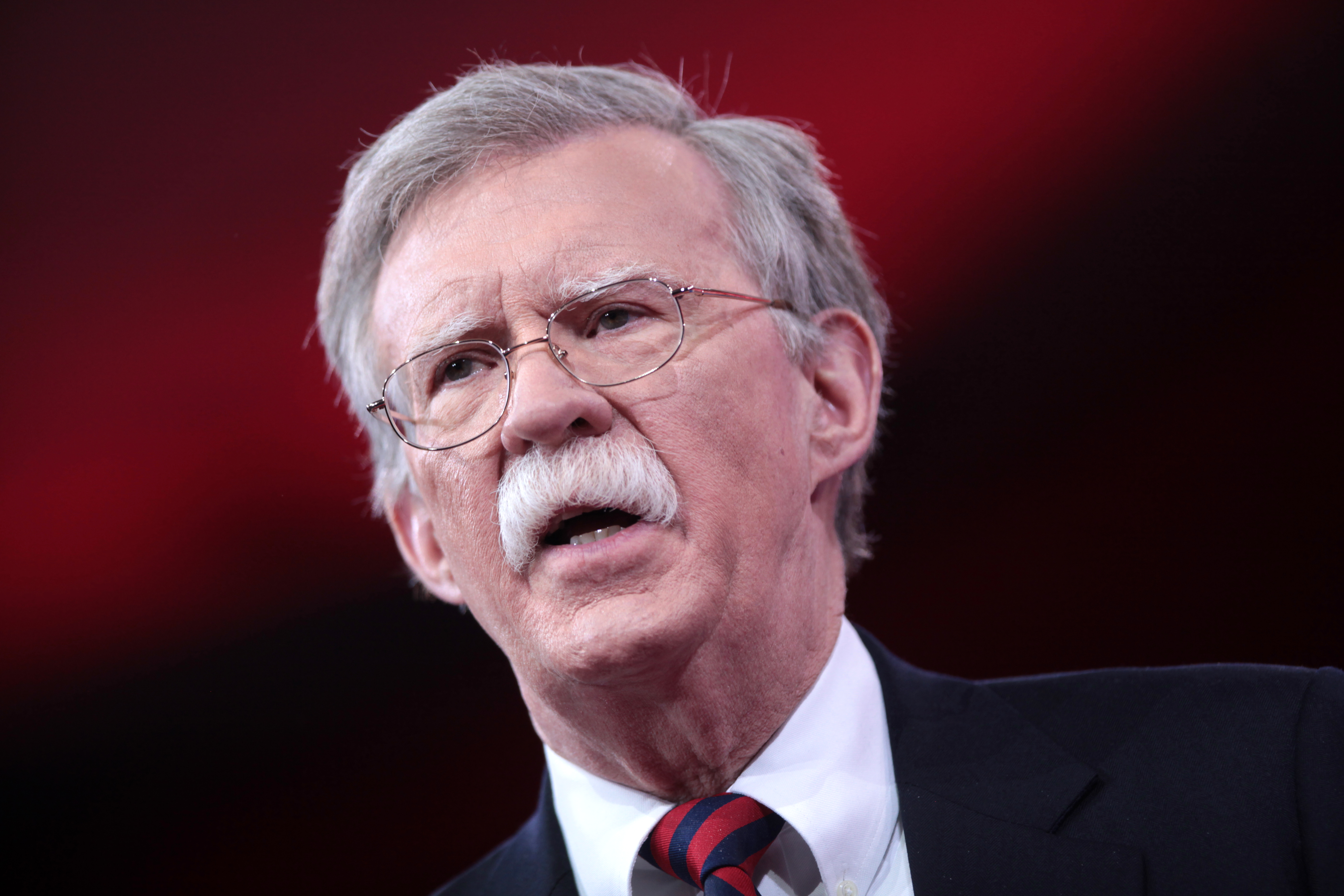The close-up photograph captures an older man, likely in his 60s or early 70s, who appears to be on stage, possibly during a speech. The background is predominantly a mix of red hues with a hint of dark maroon-brown stripe running through it. The man, positioned centrally but slightly tilted to the left, has very short, parted gray hair that slightly flops to the right, and wears thin gold metal-framed glasses. His serious green eyes look to the side and his mouth is partially open, suggesting he is about to speak. He sports a distinguished white mustache and is dressed in a dark blue suit jacket, a white shirt, and a red and navy blue striped tie. The image is cut off just below his neck, revealing only a small portion of his shoulders. The entire composition hints at a formal occasion or speaking engagement, where the man's poised demeanor and attire reflect his significant presence. Some believe his last name could be Bolton and might be associated with the Trump administration.